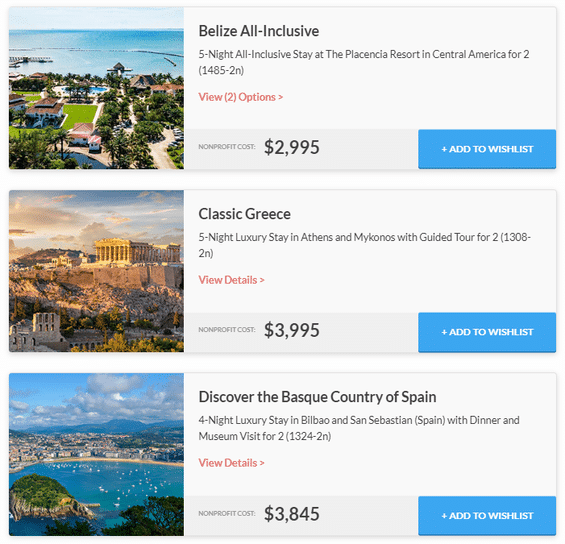The image showcases three luxurious vacation packages, each offering unique experiences in stunning locations.

1. **Belize All-Inclusive**: Enjoy a five-night all-inclusive stay at the upscale Plasencia Resort in Central America for two guests. The package is priced at $1,485 per night, with an option to view more details and an add-to-wishlist button. The non-profit cost is listed as $2,995. Accompanying the description is an inviting image of the resort area, featuring pristine ocean views, lavishly designed housing, and lush green trees, reflecting the resort's exclusive ambiance.

2. **Classic Greece**: This package offers a five-night luxury stay in Athens and Mykonos, complete with a guided tour for two. The price is $1,308 per night, and there are options to view more details and add to a wishlist. The non-profit cost for this trip is $3,995. The visual associated with this trip shows the iconic Parthenon temple and ancient Greek ruins, capturing the rich historical essence of Greece.

3. **Discover Spain**: Experience a four-night luxury stay in Bilbao and San Sebastian, Spain, which includes dinner and a museum visit for two. The cost is $1,324 per night, with available buttons for viewing details and adding to a wishlist. The non-profit cost stands at $3,845. The image for this package features a picturesque scene of Spain with a vast expanse of water, highlighting the country's scenic beauty.

Each package is designed to offer a memorable and culturally enriching experience, adorned with high-quality visuals that entice potential travelers.